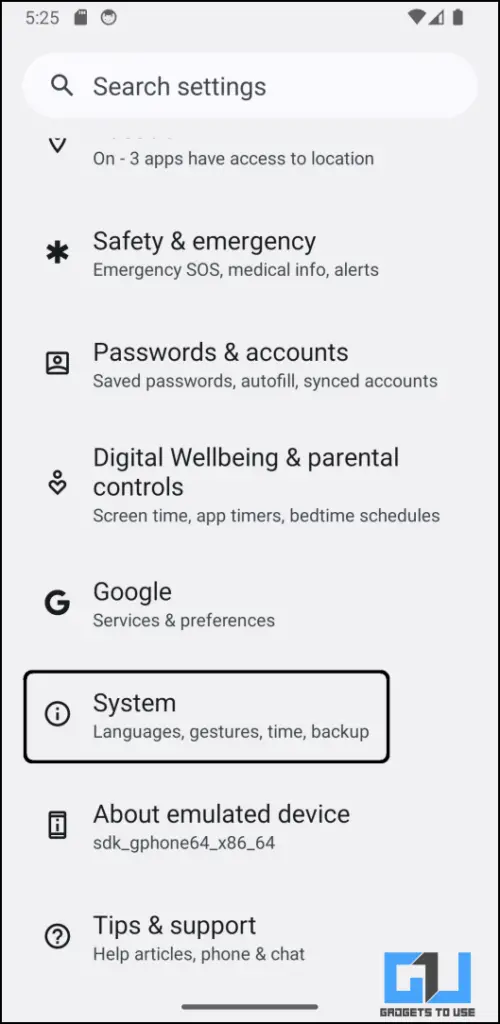A screenshot of a smartphone settings page featuring various system and app configurations. The top section displays a notification area with the time "5:25" and icons indicating full cell signal, Wi-Fi connectivity, and a fully charged battery. Below this, a search bar labeled "Search settings" is present for user convenience.

The settings menu lists several options: three apps with access to Location, Safety & Emergency settings including Emergency SOS, Medical Info, and Alerts. It also features sections such as Passwords & Accounts with Saved Passwords and Autofill, Sync Accounts, Digital Well-being & Parental Controls (comprising Screen Time, App Timers, and Bedtime Schedules), and Google Services & Preferences. Additionally, there is a detailed System section encompassing Language, Gestures, Time, and Backup, which is highlighted and marked by a black rectangle.

Further down, an emulated device identifier “sdk_gphone64_x86_64” is displayed, followed by sections for Tips & Support with Help Articles, and options for Phone and Chat support. Situated at the bottom right corner is an icon beside the text "Grommets to use," with a logo in blue and black hues.

The overall theme of the page is minimalist, with a gray background and black font, accented by blue and white highlights.